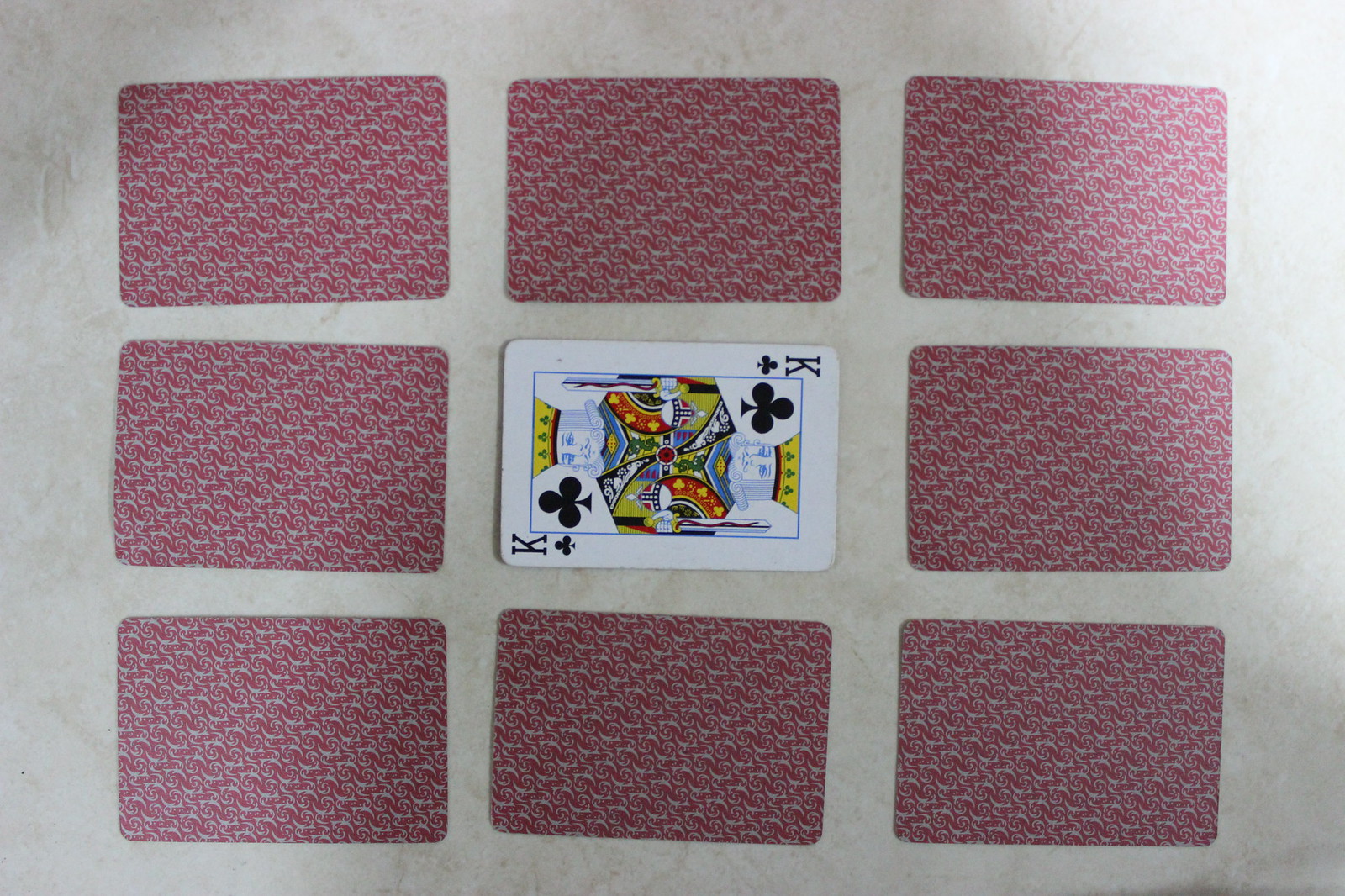A grid of nine poker cards is carefully arranged in a 3x3 layout on a light grey granite surface. The arrangement features eight cards face down, while the central card is the King of Clubs, displaying its intricate, symmetrical design with mirror image kings at the top and bottom. The cards, standard in appearance without any unusual designs, are oriented sideways, suggesting either an intentional artistic choice or a rotated picture. The overall scene captures a moment that hints at either an underlying game or an aesthetic presentation.